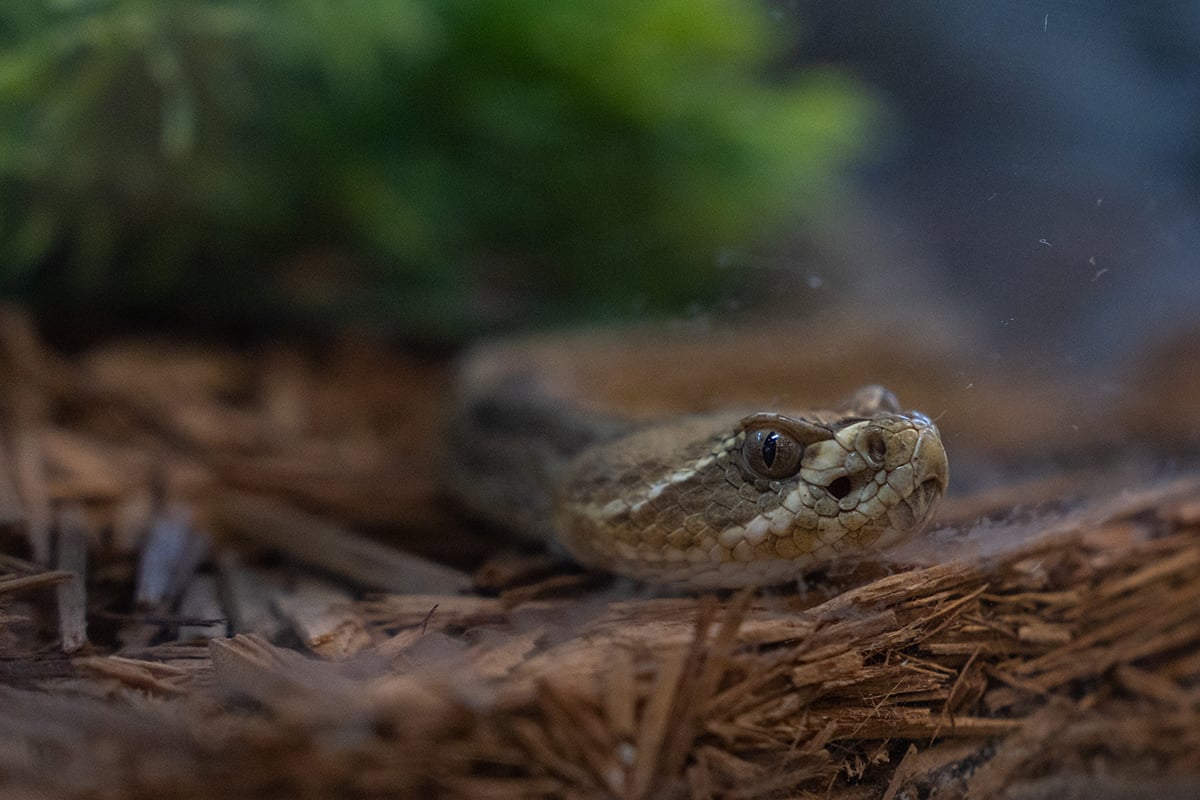This close-up image captures the intense gaze of a rattlesnake, positioned prominently in the center of the frame. The snake's head, seemingly looking to the right, exudes a fearsome presence with its distinct, lizard-like features. Its eyes are spherical, dark brown with black pupils, contributing to its intimidating look. The background, though blurry, allows the detailed textures of the rattlesnake's head to stand out. The scales on its face are finely detailed, presenting a blend of light cream and dark brown colors, which help it blend seamlessly with its surroundings. The ground beneath is a mix of scattered wood debris, enhancing the snake's natural camouflage. The blurred backdrop includes additional pieces of wood and a large green bush in the upper left corner, providing a contrasting splash of color to the earthy tones of the rattlesnake and its immediate vicinity.